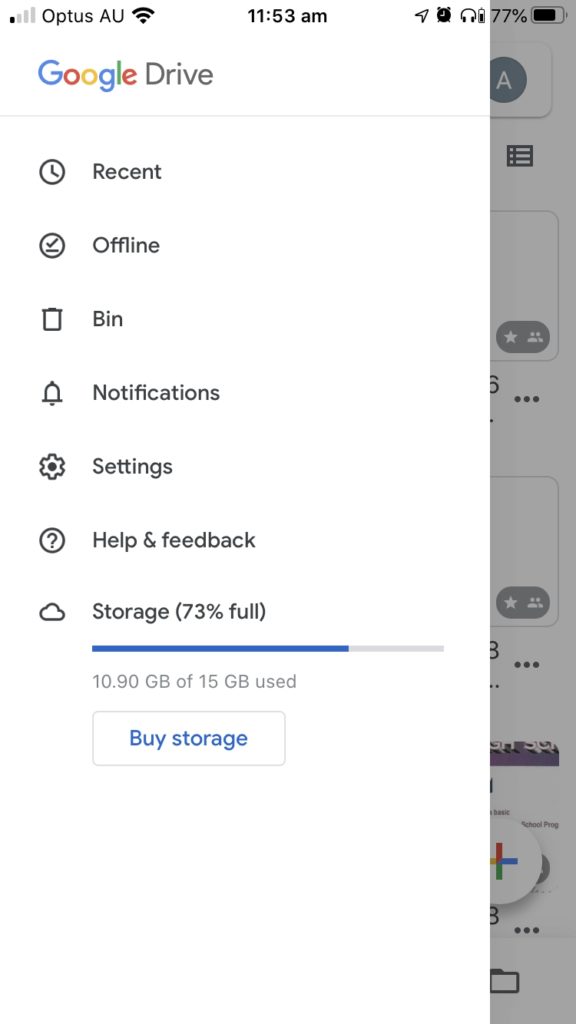This is a detailed description of a phone screenshot displaying a pop-up tab. The tab emerges from the left side of the screen, covering a portion that extends nearly to the right edge, casting a shadow over the right part of the display. Within this shaded area, at the top right corner, the screen shows a battery percentage of "77%" and an icon of a phone in black. Below this, there is a gray circle containing a white letter "A," followed by another gray circle with three sideways exclamation points.

Further down, there is a gray tab with a star and a count icon. Another similar gray tab is located below this, and at the bottom right corner, there is a partial view of a white circle with half of a plus sign.

On the left side within the white-background pop-up, the top left corner shows full internet bars labeled "Optus, AU," followed by a Wi-Fi icon and the time "11:53 a.m." Below this, a list of items appears, each followed by matching icons. The list includes "Google" in its classic colors, "Drive," and a thin gray line separates these from the items below. The listed items further include "Recent," "Offline," "Notifications," "Settings," "Help & Feedback," "Storage 73% full," with each having corresponding icons on the left.

Beneath this list is a progress bar, mostly blue (representing 75%) with the remaining 25% in gray. Below, smaller gray text reads, "10.90 GB of 15 GB used." At the bottom, there is a white tab with a gray border and the blue text "Buy storage."